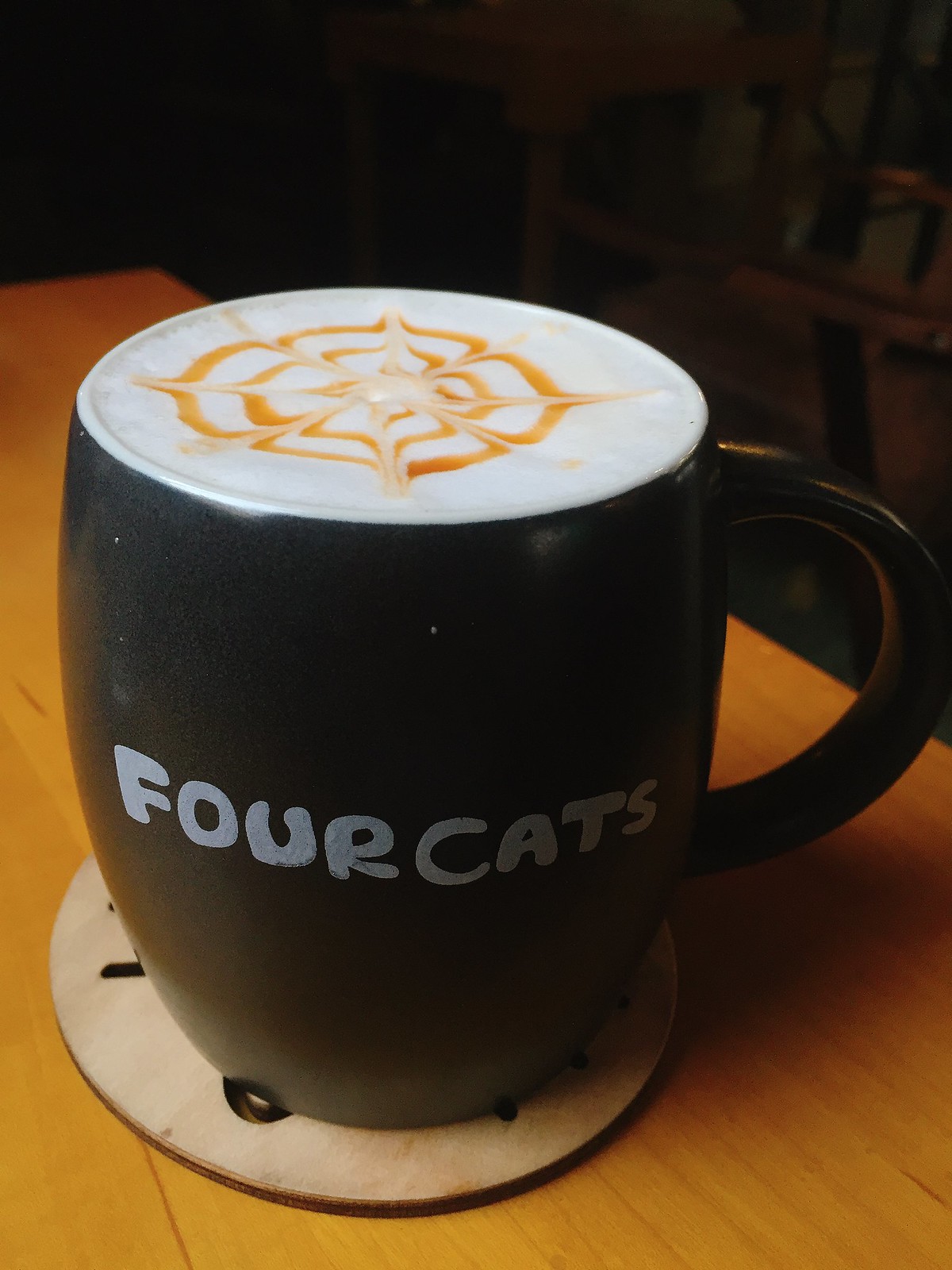This is a close-up, color photograph of a black coffee mug with a black handle, sitting on a golden-colored wooden table atop a lighter wood, circular coaster. The focal point of the image is the frothy white top of the coffee, adorned with an intricate, caramel-colored pattern that resembles both a star and a flower with eight petals. This artistic design, likely created using milk and coffee, gives the impression of a detailed latte art piece. Across the front of the mug, in a playful, cartoonish white font, are the words "For Cats." The lighting in the room is low and comes from the bottom left corner, giving the image a moody ambiance. The background is dark and blurry, suggesting the setting is possibly a barista’s counter or coffee shop, adding to the intimate feel of the scene.